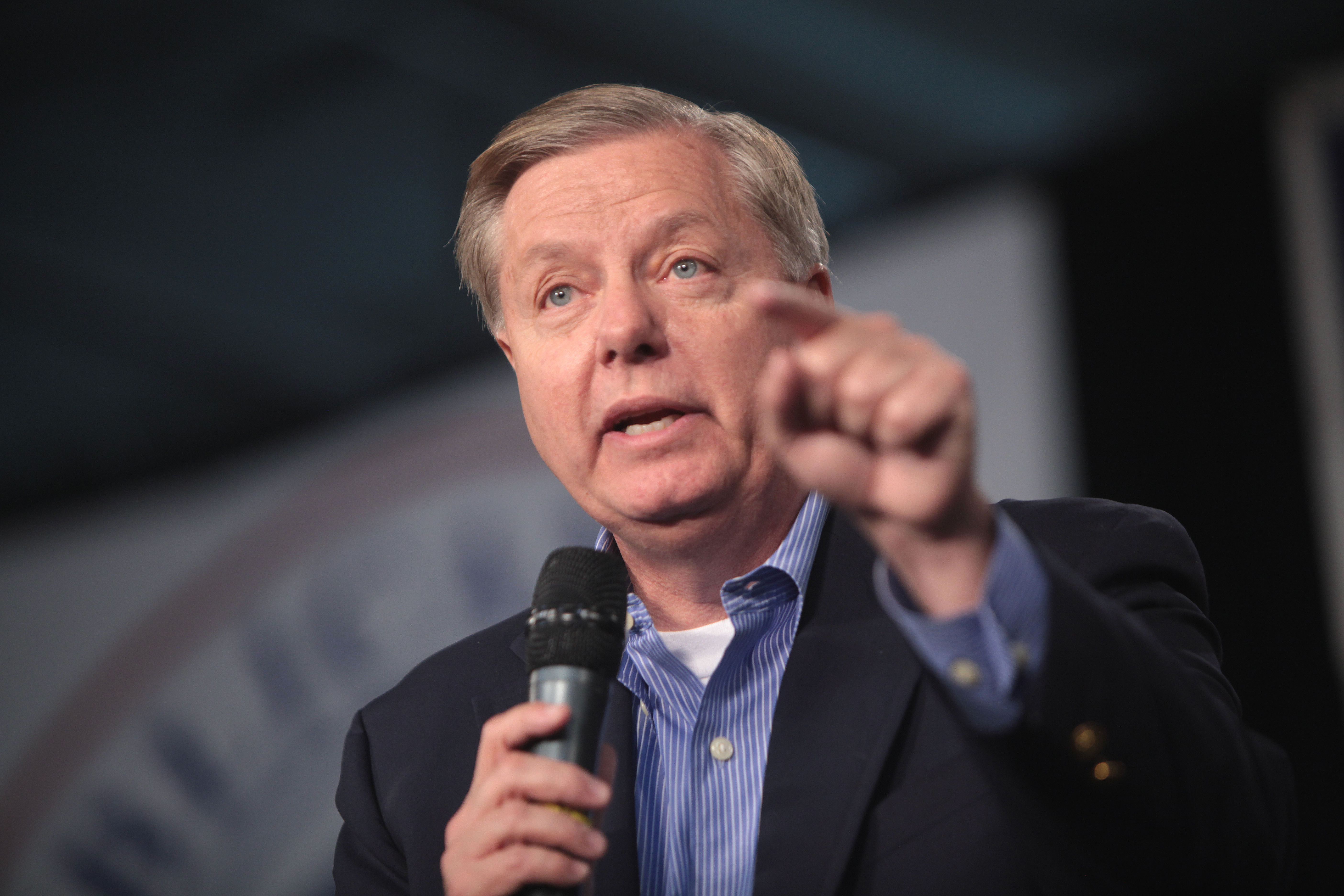This image captures an indoor event featuring a politician, likely U.S. congressman McCarthy, who appears to be in his mid-60s. He is speaking into a microphone held in his right hand, while his left hand is pointed accusatorily at someone, possibly indicating a moment of intensity or upset. The man is dressed in a blue blazer over a blue and white striped button-down shirt, which is partially unbuttoned at the collar, revealing a white t-shirt underneath. He has gray, light-brown hair combed to the side, pale skin, and blue eyes. The background is blurred but shows hints of blues and grays towards the top, a light-colored wall with an indistinct blue image or seal, and a dark ceiling. The overall scene suggests a formal indoor setting with an engaged audience.